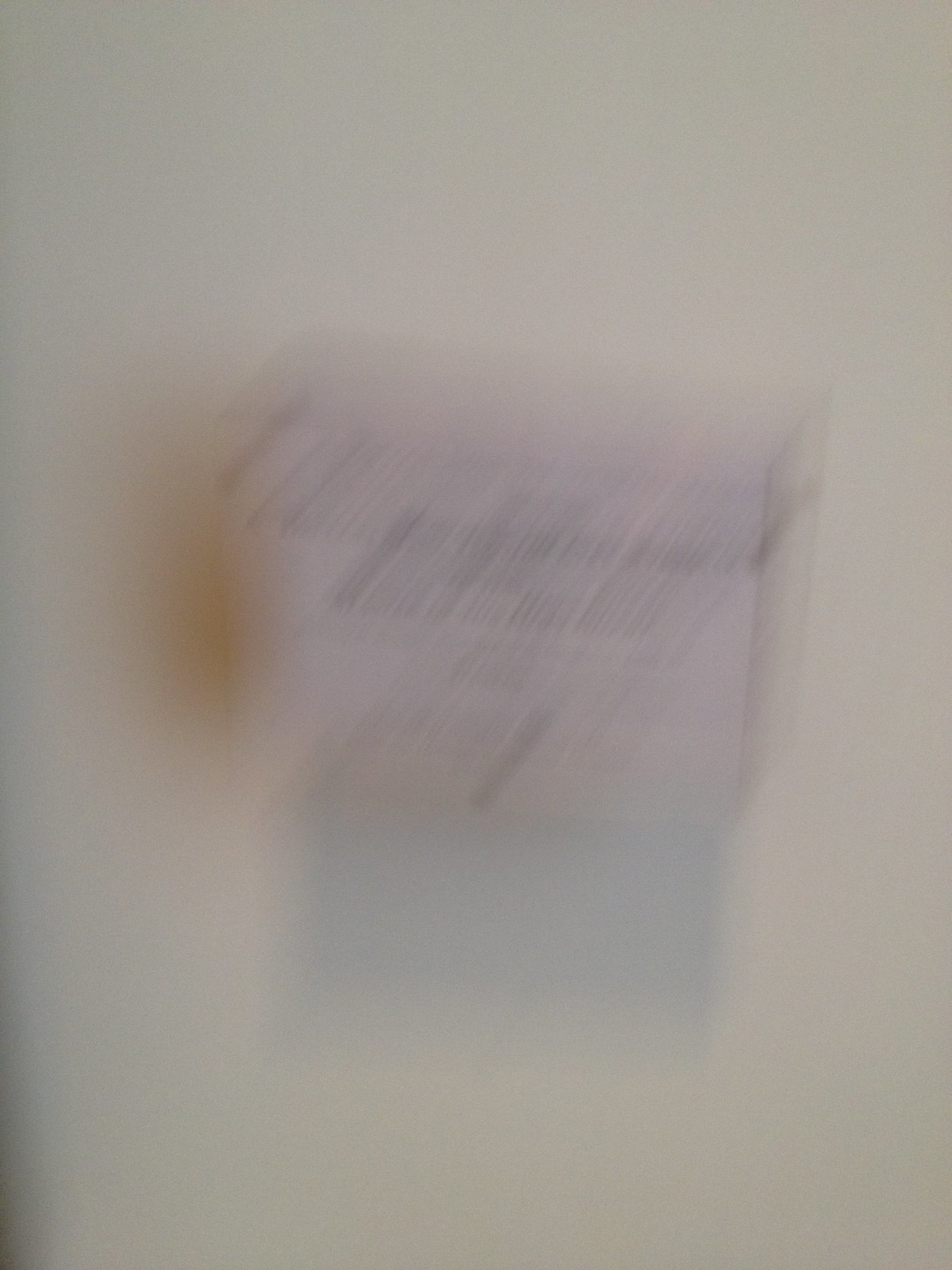A very blurry image depicts what appears to be a piece of paper hanging on a white wall. The paper, with a landscape orientation, resembles an award due to its layout. At the top, there's cursive writing in black ink, followed by several lines of smaller text. On the left-hand side of the paper, there is a yellowish splotch of something indiscernible. Beneath the paper, a light blue area can be seen, but its purpose is unclear due to the overall blurriness of the image.